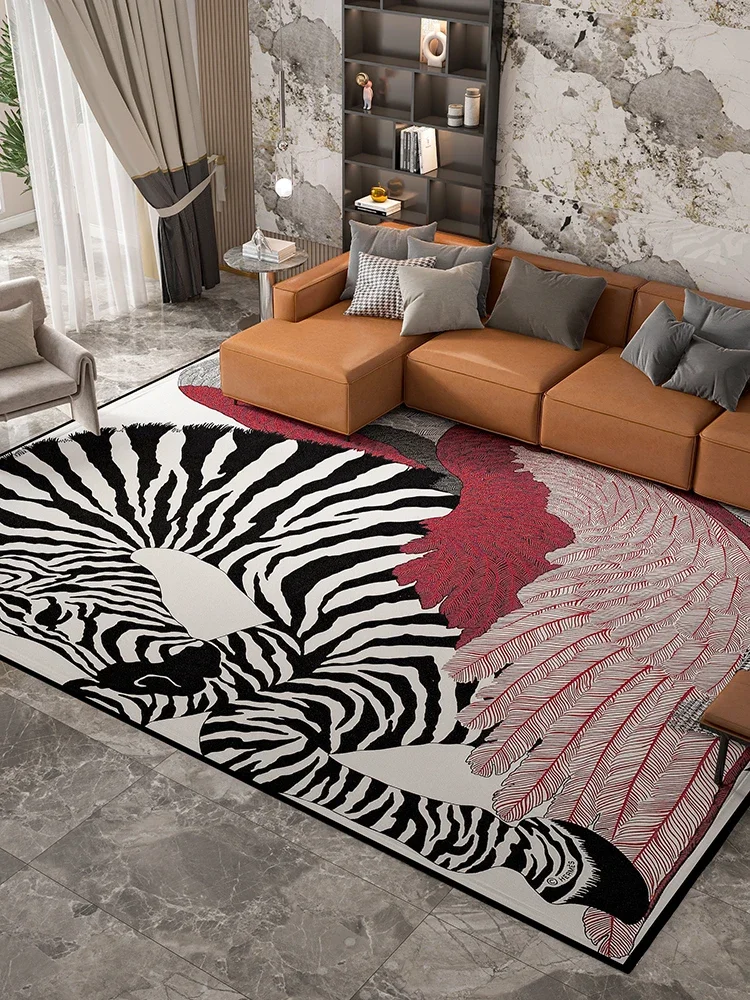This image showcases a modern living room with a focus on a unique area rug as the centerpiece. The room features gray granite or marble floors, complemented by distressed or exposed brick-like wallpaper, giving it a rustic yet contemporary feel. A large window or door is adorned with open curtains, allowing ample natural light to flood the space.

Dominating the room is a striking area rug that captures immediate attention. The rug's design depicts a zebra in a lying-down position with its forelegs stretched out and its head down. The zebra is partially covered by large, vivid red and pink feathers, creating a visually arresting graphic. 

A brownish-tan leather sectional sofa with a chaise lounge end faces the rug, outfitted with numerous gray throw pillows scattered across it. Behind the sofa stands a bookcase, adding a touch of functionality to the room. Overall, the space harmoniously blends modern and rustic elements, creating a stylish and inviting atmosphere.